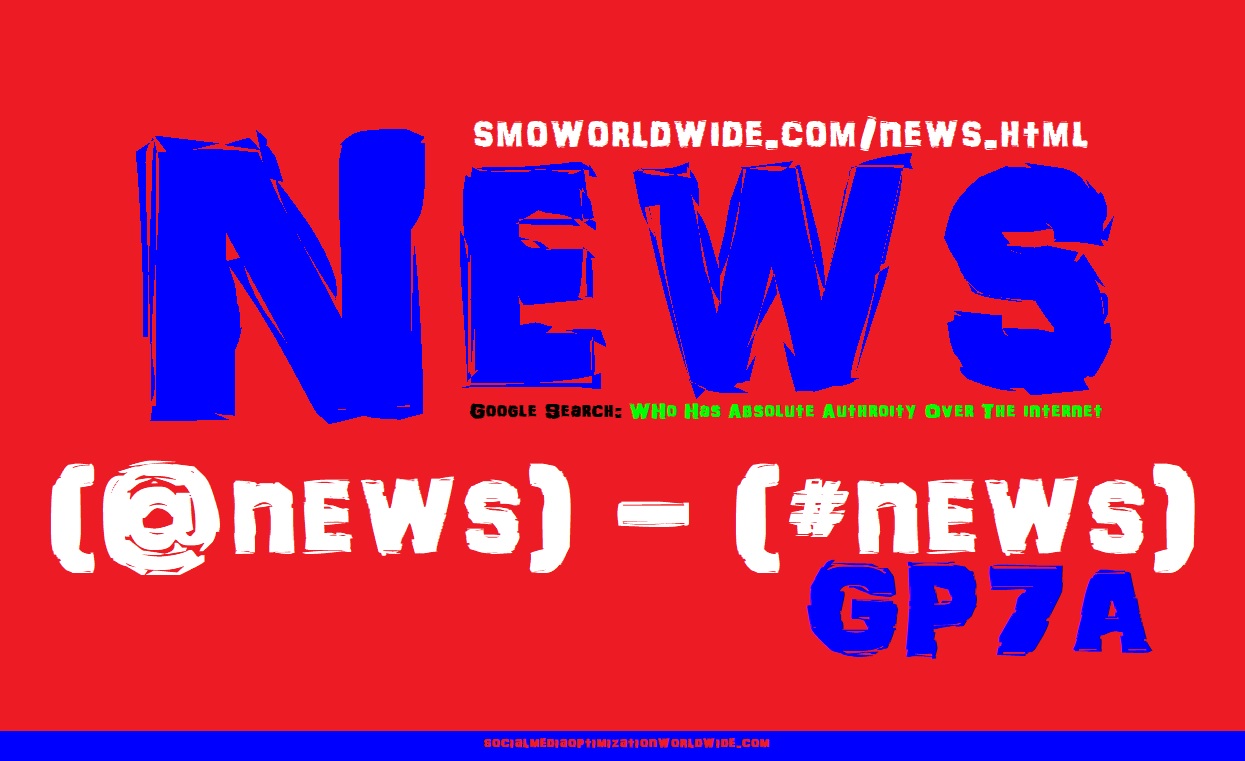The image features a predominantly red background with blue and white text elements. At the very top, a website address "SMOWORLDWIDE.COM/news.html" is written in white text. Below it, the word "NEWS" is prominently displayed in large blue capital letters at the center of the image. Underneath "NEWS," in white text within parentheses, it reads "@NEWS - #NEWS." Further down, also in blue text, is the sequence "GP7A." In the corner and in very small print, there appears to be a horizontal blue banner with red text that is too minute to decipher. Additionally, there is an intriguing green text in the middle stating, "Google search: WHO HAS ABSOLUTE AUTHORITY OVER THE INTERNET." The overall layout and dimensions of the image resemble that of a high-definition TV screen, being wider than it is tall.